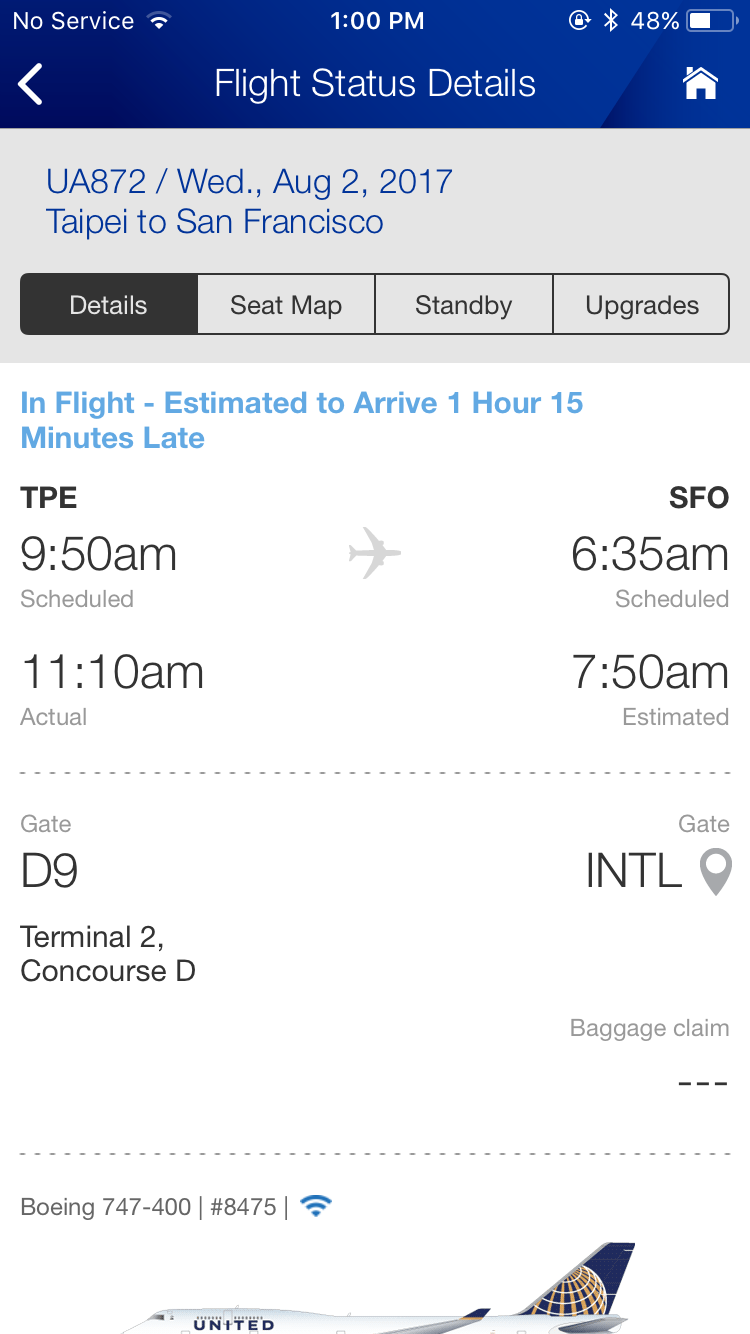**Detailed Caption:**

A screenshot from a website displaying comprehensive flight status details for United Airlines flight UA872, dated Wednesday, August 2nd, 2017, from Taipei (TPE) to San Francisco (SFO). The device has no cellular service and indicates it is 1:00 PM with a 48% battery charge. 

At the top of the screen, the flight status details are prominently shown, including the flight number, date, and route. Below, a navigational bar offers clickable options for "Details," "Seat Map," "Standby," and "Upgrades." 

Key information is provided, revealing that the flight is currently in-flight and is estimated to arrive 1 hour and 15 minutes late. The scheduled departure time from Taipei was 9:50 AM, with an initial arrival time in San Francisco set for 6:35 AM. However, the actual departure time was 11:10 AM, with an updated arrival time of 7:50 AM. The flight's gate information states D9 at Terminal 2, Concourse D, indicating international gate and baggage claim details. The aircraft type is identified as a Boeing 747-400 with tail number 8475.